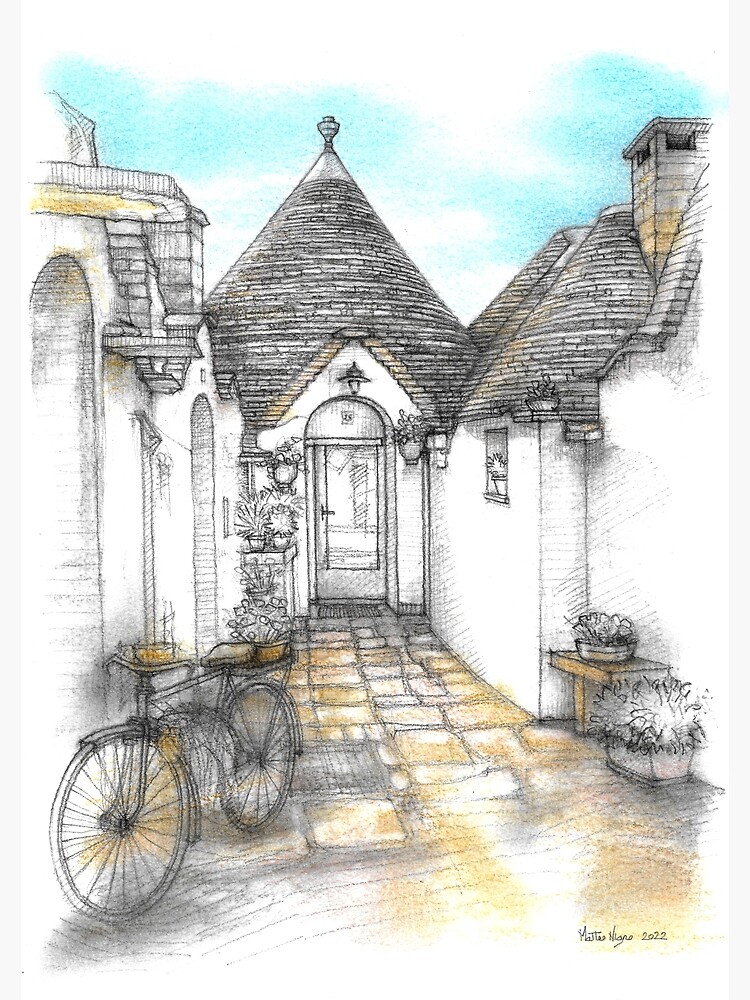This detailed pencil and ink drawing, signed in 2022, portrays a charming courtyard scene accented with watercolor hues of yellow, blue, brown, and gray. The composition features an old-fashioned, multi-spoke bicycle with a flower-filled basket situated on the yellow and gray cobblestone street in the front left. To the right, a yellow-tan table holds a pot of flowers, and beside it stands a planter with a bushy plant. The courtyard is framed by white stone buildings with steep, tiled or shingled peaked roofs, one of which has a chimney. At the center is an arched doorway leading into a building, adorned with an ornate chalice-shaped object atop the roof. The background sky is lightly rendered in blue with scattered clouds.